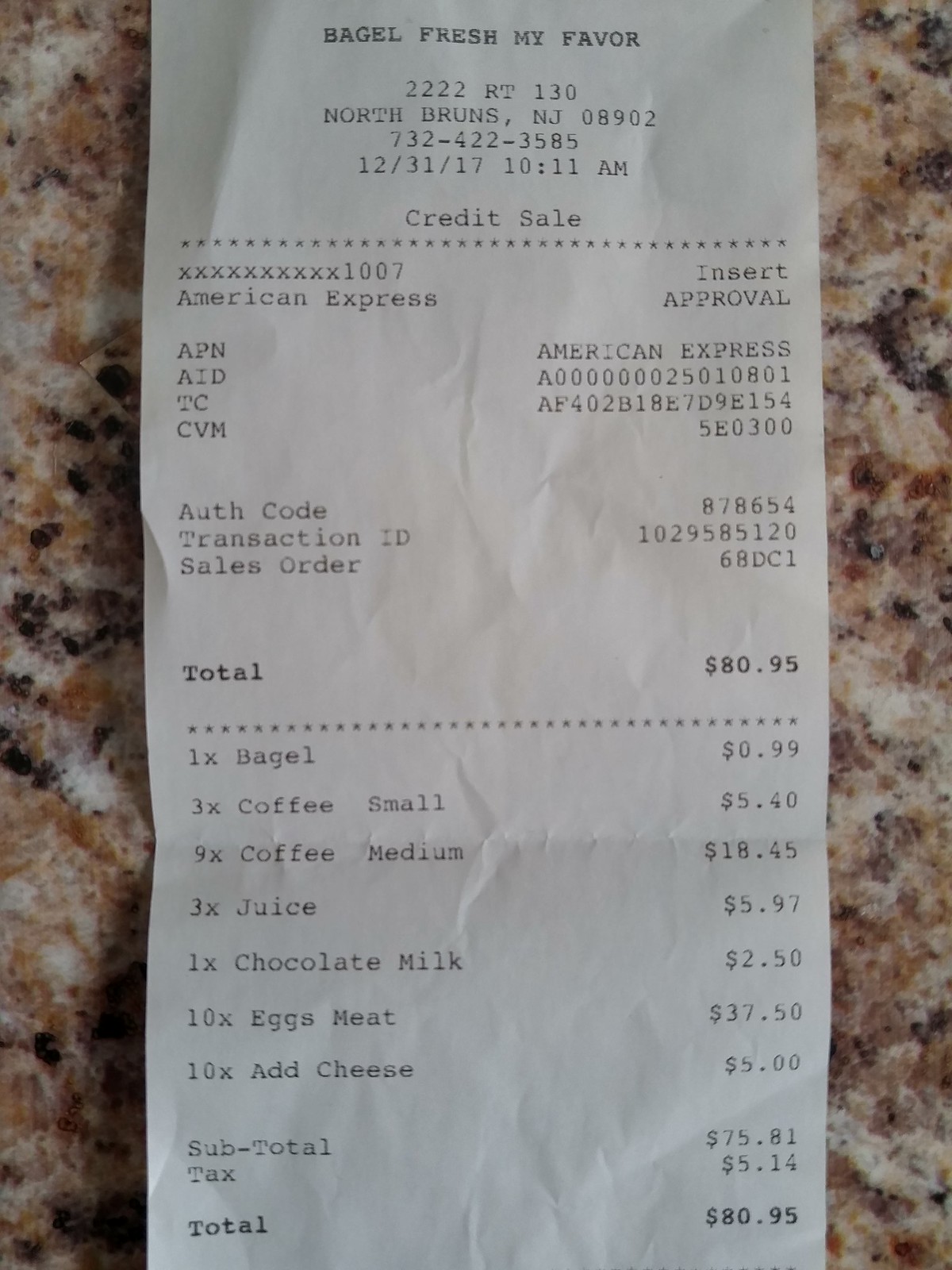This photograph showcases an up-close image of a white receipt from "Bagel Fresh My Favor," nestled on a brown and black speckled granite or marble countertop. The receipt details a purchase made at 2222 Route 130, North Bronx, New Jersey 08902, on December 31st, 2017, at 10:11 AM via credit sale using American Express. The total amount is prominently displayed as $80.95. A breakdown of the purchased items includes one bagel for $0.99, three small coffees for $5.40, nine medium coffees for $18.45, three juices for $5.97, one chocolate milk for $2.50, ten eggs with meat for $37.50, and ten additional slices of cheese for $5.00. The receipt also features transaction details such as an authorization code and a sales order ID labeled 68DC1.